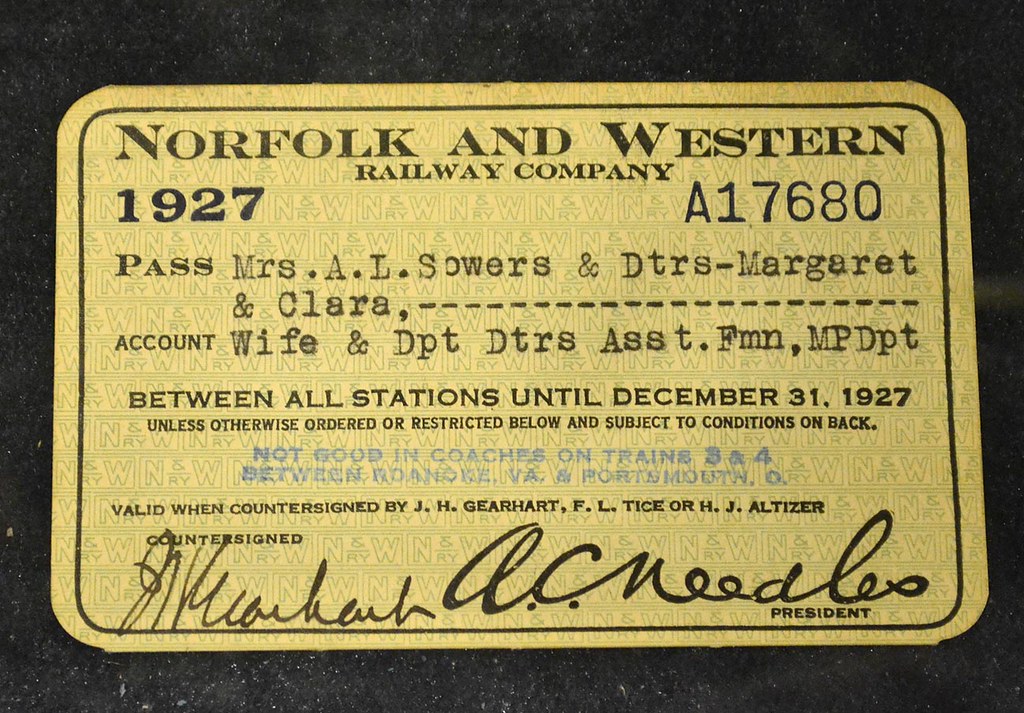The image depicts a golden ticket, reminiscent of a historical railway pass, placed on a sleek black surface, possibly a quartz countertop or table. The card, approximately the size of a credit card, features rounded corners and a striking black border. Dominating the top of the ticket, bold black text reads: "Norfolk and Western Railway Company, 1927," with the serial number "A17680" prominently displayed to the right. Below this header, the ticket is marked as a "PASS" and elaborately details the names "Mrs. A.L. Sowers and DTRS Margaret and Clara," noting their relation "Account Wife and Department DTRS Assistant FMN MPD PT." The pass grants travel "Between All Stations until December 31, 1927, unless otherwise ordered or restricted below and subject to conditions on back."

A distinctive blue stamp cautions, "Not Good in Coaches on Trains 3 and 4 between Roanoke, VA and Portsmouth, O." The ticket also specifies it is valid only when countersigned by "J.H. Gearhart, F.L. Tice, or H.J. Althyser," with space for a cursive signature at the bottom. Further enhancing its vintage authenticity, the ticket’s background features a repeating pattern of the letters "N&W."